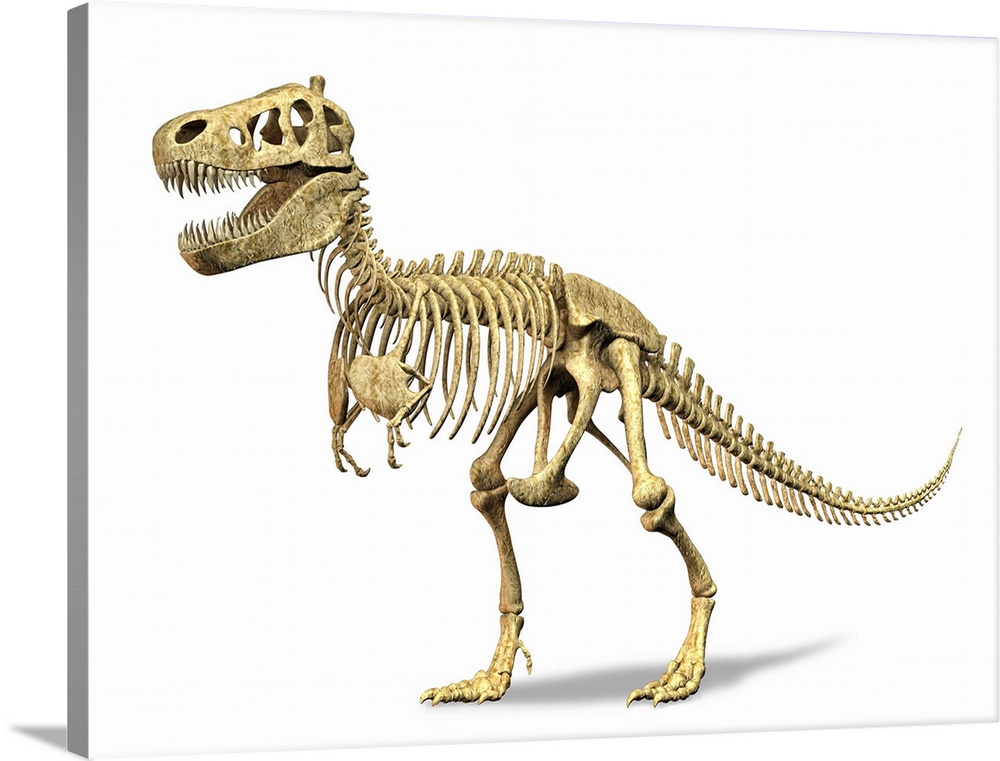This image depicts a detailed skeleton of a Tyrannosaurus Rex, prominently displayed on a thick, white, canvas-like box that provides a sense of depth and casts a slight shadow. The T-Rex skeleton is positioned as if in motion, walking on its sturdy hind legs, with its right leg stepping forward. It faces left, showcasing its massive skull with an open mouth filled with sharp teeth. The skeletal structure reveals a long, outstretched tail extending to the right side of the frame, while the spine runs seamlessly from the skull down to the tail. The dinosaur’s small, claw-like front limbs dangle in front of its chest. The skeleton is tan with darker shading in areas like the groin and back feet, giving it a more three-dimensional appearance. The image, which appears digitalized, emphasizes the intricate details of the bones and the T-Rex's imposing stature against the stark white background.